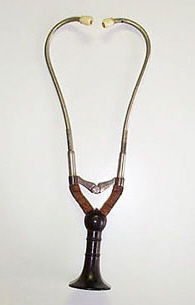This image depicts a vintage stethoscope placed against a light gray background. The stethoscope features white eartips, now slightly discolored to a creamy tan hue, that fit into the physician's ears. From these eartips, curved metal tubes extend downwards, converging into a connection point secured by a piece of beige-orange textile. This section leads into the stethoscope's iconic chest piece. The lower part, resembling a trumpet or horn, appears to be made of dark brown metal or black material, which would be placed against the patient's chest for auscultation. The device’s age is evident from its materials and design, which differ significantly from modern stethoscopes.